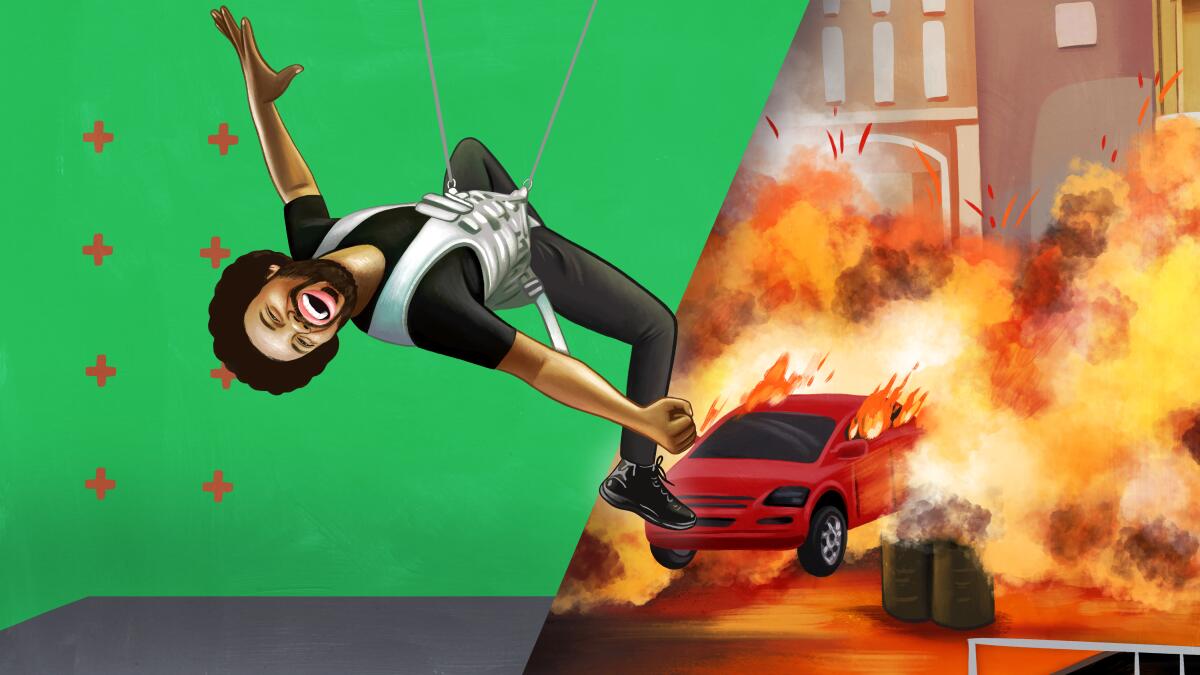The image is a detailed digital illustration, seemingly from a wikiHow article on becoming a stuntman or stuntwoman. It is divided diagonally into two distinct scenes. On the left, a man with an afro, laughing and suspended upside down by a harness rigged to wires, is set against a lime green screen background with gray flooring. Red crosshair markings are visible, indicating positioning points. This setup suggests he's simulating being blown away. The right side transitions dramatically into a vibrant, animated scene: a flaming sedan in front of a building, engulfed in fire from an explosion. The stark contrast between the practical setup and the fiery, final shot emphasizes the transformation from behind-the-scenes stunt work to the finished, action-packed spectacle.